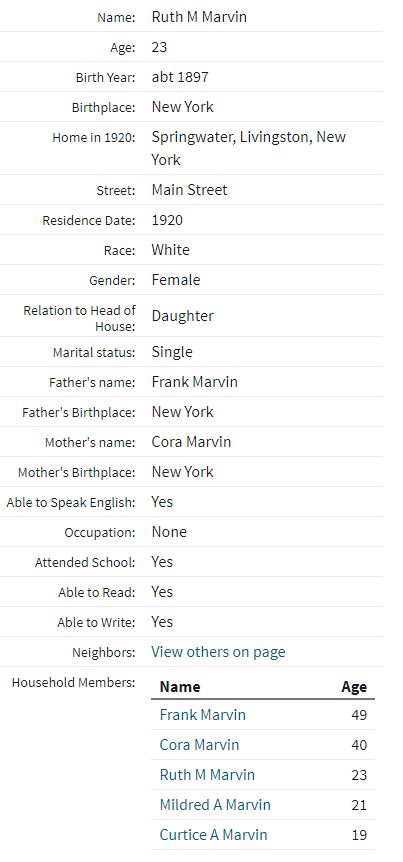The image depicts a detailed record from a census page on a genealogy website, characterized by its white background and neatly organized information presented in light blue and black fonts. The primary individual featured is Ruth M. Marvin, born around 1897, making her 23 years old at the time of the record. Her birthplace is New York, and her residence in 1920 was at Main Street in Springwater, Livingston, New York. The record indicates her race as white, her gender as female, and notes her as being the daughter in the household, with a marital status of single. 

Additional demographics include her parents: Frank Marvin, age 49, and Cora Marvin, age 40, both listed with New York as their birthplace. Other household members include Ruth's siblings, Mildred Marvin, 21, and Curtis A. Marvin, 19. Ruth is identified as able to speak English, read, and write, though she had no occupation at the time but did attend school. This meticulously compiled data provides a comprehensive snapshot of the Marvin family's composition and status as recorded in the 1920 census.